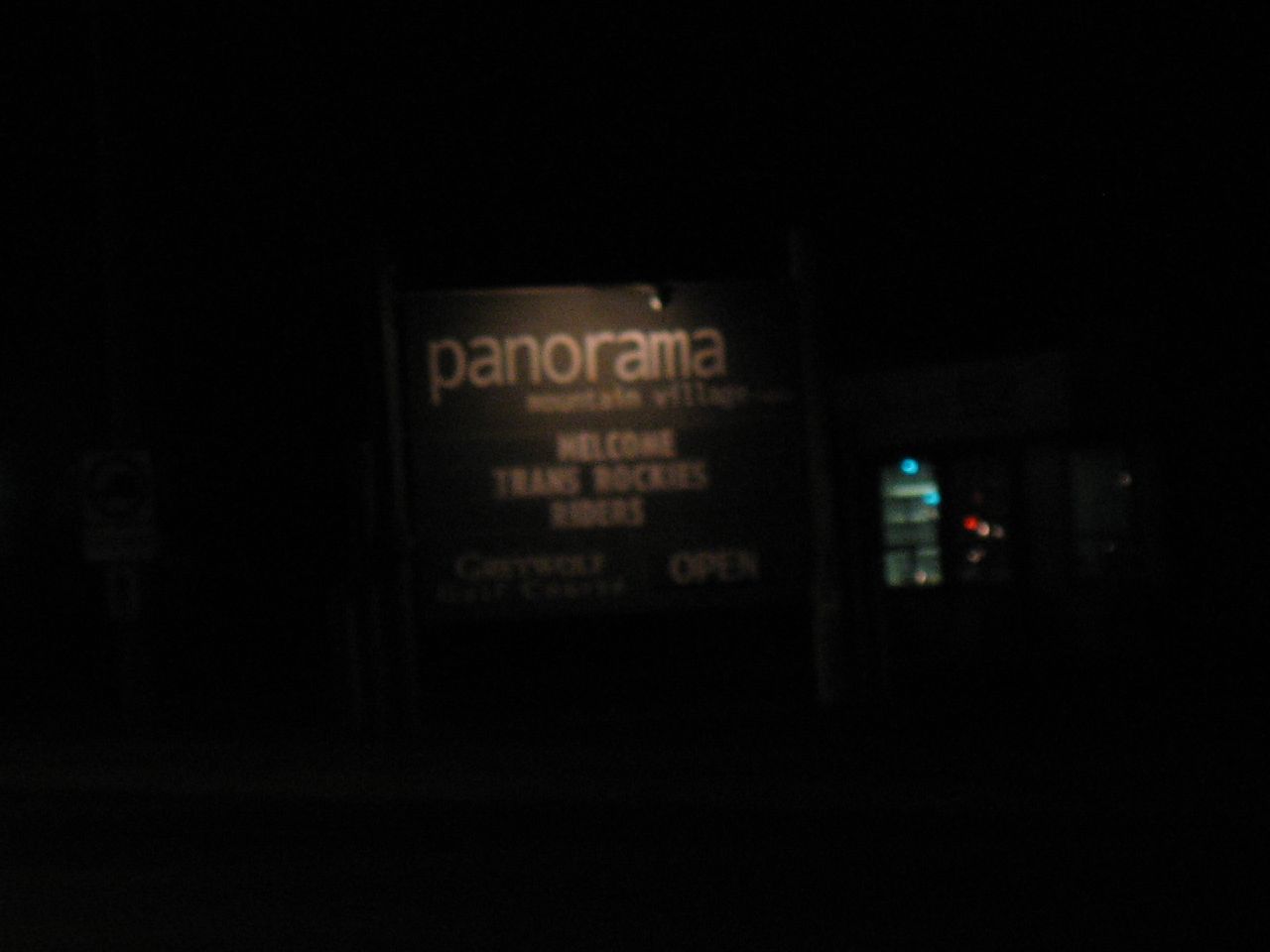This nighttime photograph captures a dark and grainy image of a sign that reads "Panorama Mountain Village," with the words "WELCOME TRANS ROCKETS WRITERS" in bold capital letters beneath it. The lower left portion of the sign contains illegible text due to the lack of light. The overall quality of the image is low, making it appear somewhat blurry. In the bottom right corner, the word "OPEN" is prominently displayed in all capital letters, likely in white or another light color against the dark background of the sign. The sign is illuminated by a small light fixture that extends outwards. To the right of the sign, there's a very indistinct and fuzzy area that might depict city life, but the details are lost in the darkness. Some blue and red lights are also faintly visible, possibly belonging to traffic or vehicles, though their shapes are not discernible. The predominant feature of the photograph is the sign, set against an otherwise nearly black backdrop.